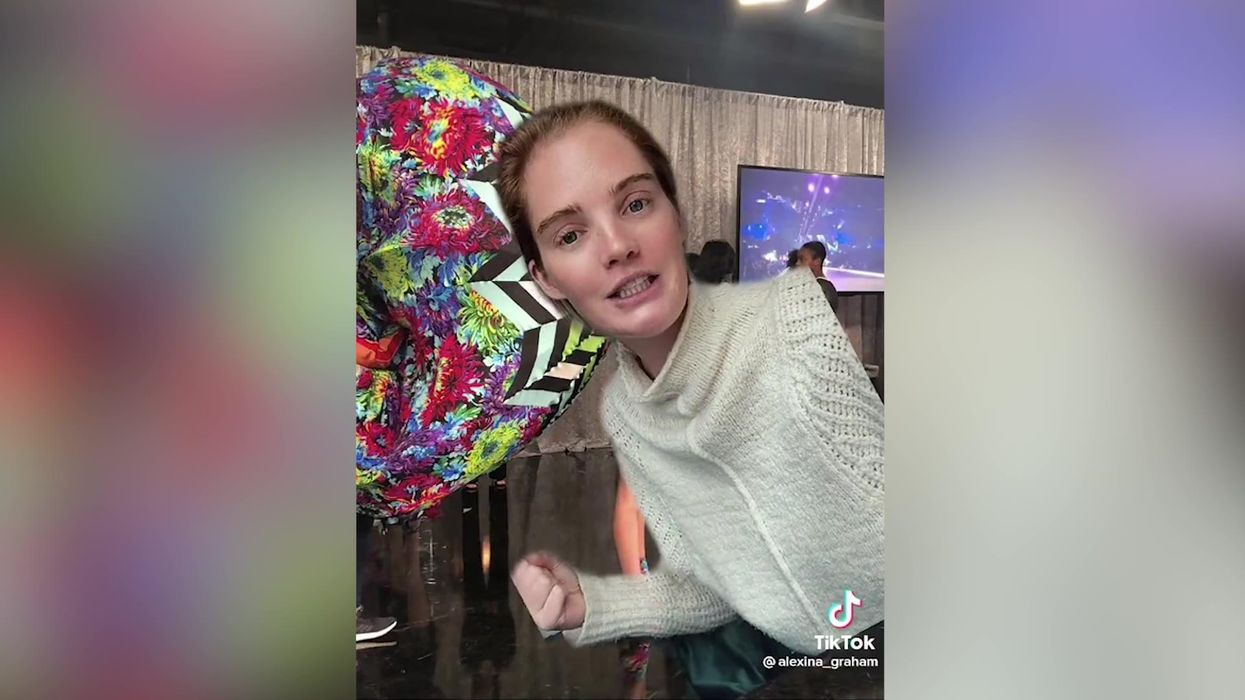This photographic image captures a close-up of a young white woman from a TikTok video, tagged at the bottom right with "TikTok @Alexina_Graham." The woman, Alexina Graham, has short brown hair, styled around her ears, and she's looking directly at the camera with her mouth slightly open. She’s wearing a long-sleeved white sweater, her right hand clenched into a fist as though poised for action. She seems to be situated indoors, possibly in a convention room or a restaurant, with parts of the environment intricately detailed. 

To her left is a distinctive balloon adorned with red flowers and black-and-white chevron patterns, adding a splash of color to the background. Behind her, a curtain can be seen, separating the setting into defined spaces. In front of the curtain, there is a television screen and a group of three people sitting, one of whom appears to be black. The wide array of colors and objects around her, though somewhat blurred and ambiguous, suggest a vibrant setting possibly altered or enhanced digitally, with elements like the large, colorful object to the far left contributing to an almost surreal atmosphere.